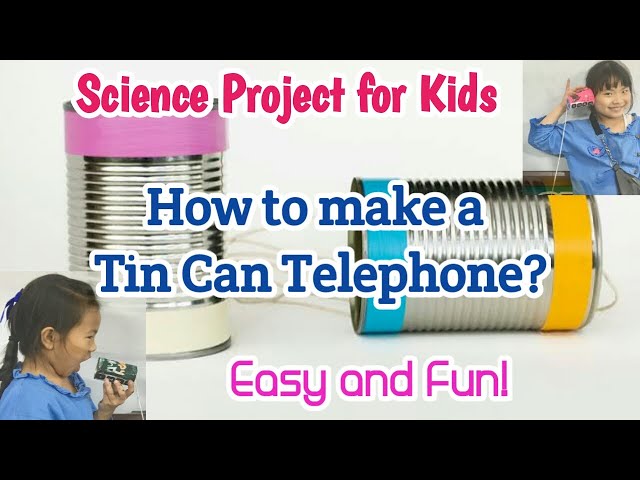This is a detailed photograph featuring instructions titled "Science Project for Kids: How to Make a Tin Can Telephone," set against a lighter backdrop bordered with black bars at the top and bottom. The top red text states "Science Project for Kids," followed by blue text in the center that says "How to Make a Tin Can Telephone." The bottom section has purple text reading "Easy and Fun."

The image prominently features two Asian girls. In the bottom left corner, a girl with braided hair, adorned with a blue ribbon, is facing right and speaking into a tin can. She is dressed in a blue ruffled shirt. In the top right corner, another girl, also wearing a blue shirt, holds a pink tin can up to her ear with her right hand while smiling, with her right index finger pointing up. The central part of the image shows a pair of tin cans connected by a string, one standing upright with a pink top and the other lying on its side featuring blue and yellow ends decorated with colorful stripes. This visually engaging and instructional image effectively combines fun and educational elements, capturing the essence of a simple science project for kids.